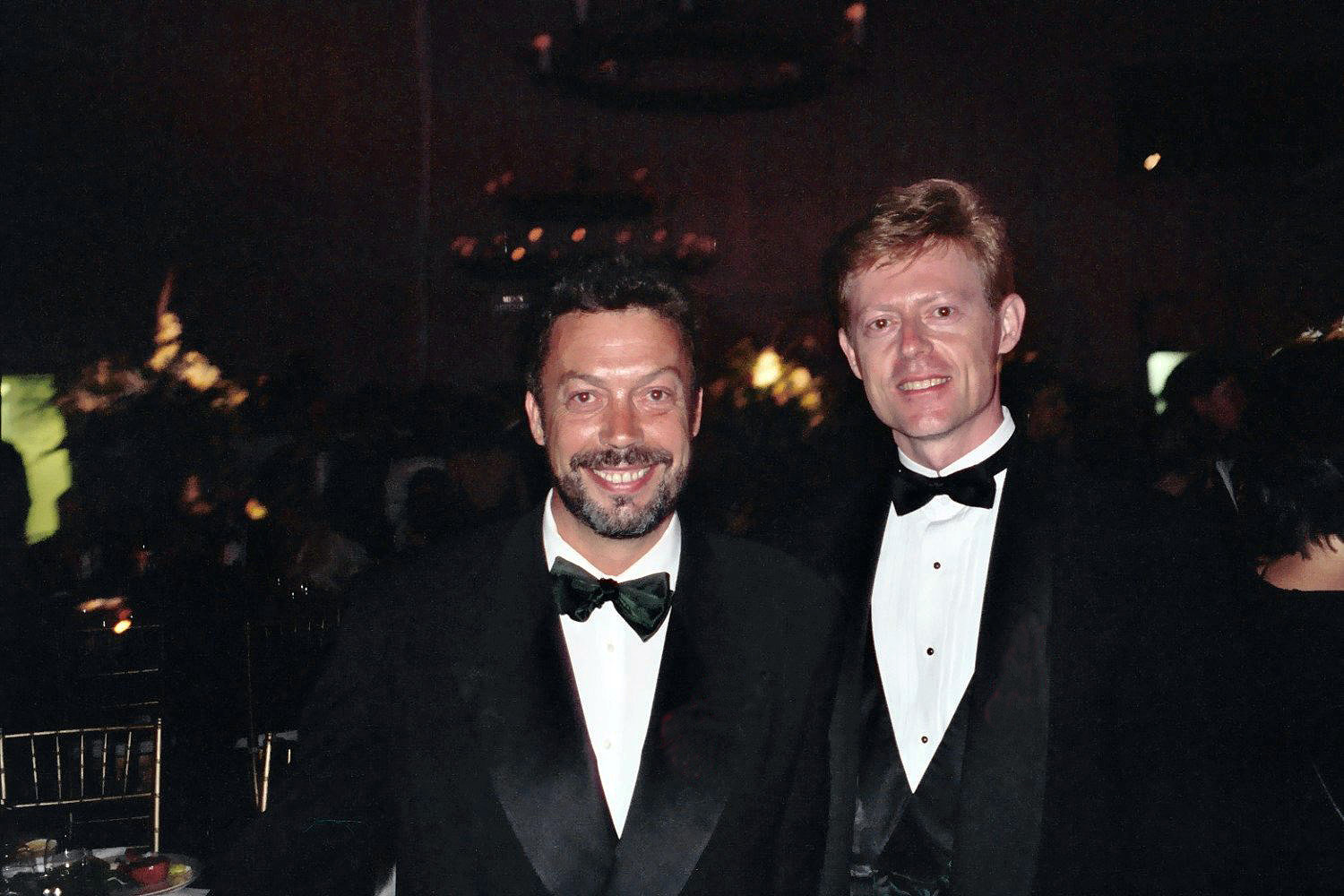In this image, two men are captured in an elegant setting, both donned in black tuxedos with matching black bow ties and white shirts. The man on the left is shorter, with dark hair, a mustache, and a beard, and his shirt features light-colored, almost invisible buttons. The taller man on the right, several inches taller, has brown hair and a clean-shaven face, his shirt distinguished by its prominent black buttons. The background is fairly dark, but illuminated by some lights, revealing chairs and a table topped with food, likely indicating a social event. A crowd is visible in the background, suggesting this may be an award show or film premiere. The man on the left might be an actor known for roles in "Legend" and "Home Alone 2," while the identity of the man on the right remains uncertain, though both exude sophistication and style.